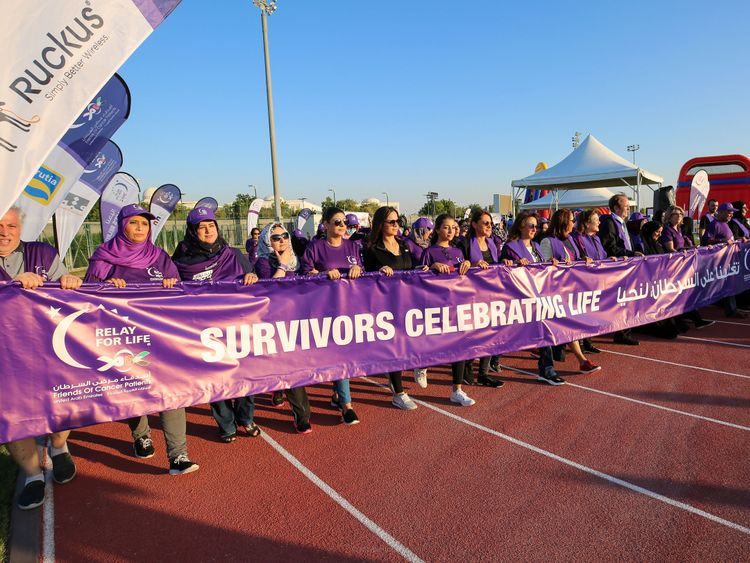In this outdoor image, a group of approximately 20 people, mostly women and some men, are standing in a line on a pinkish-red track with white stripes. They are holding a long purple banner that prominently displays "Relay for Life" on the left, "Survivors Celebrating Life" in white block letters in the center, and text in a foreign language on the right. Many participants are dressed in purple, including shirts, scarves, shawls, and hats adorned with the Relay for Life logo, featuring a crescent moon and star. Notably, one woman in the center is dressed in black, and a man on the right is donning a suit jacket with a shirt. The backdrop includes a clear blue sky with a light pole slightly left-of-center, a white tent with a triangular top, and a red object that might be a bounce house. Some women wearing hijabs hint at a diverse group, possibly including Pakistani or Middle Eastern participants. Flags for various companies, including one that reads "Ruckus, Simply Better Wireless," are visible, suggesting an organized event likely for the entire day.